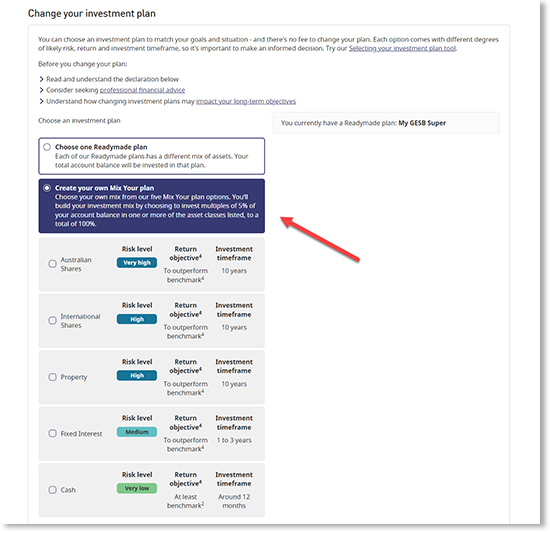The image is a detailed guide on selecting and changing investment plans, prominently titled "Change Your Investment Plan" at the top. It emphasizes the flexibility to align investment choices with individual goals and circumstances, noting there is no fee to change plans. Each investment option varies in terms of risk, expected returns, and timeframes.

Highlighted in blue text is an interactive link labeled "Try Our Selecting Your Investment Plan Tool," which suggests access to additional resources for making an informed decision. Below this, a cautionary statement advises users to read and understand their declaration before making any changes and to consider professional financial advice, emphasizing the potential long-term impact of their choices.

The current selection is a pre-constructed plan labeled "My GESB Super." Users are presented with two main options: "Choose One Ready-Made Plan" and "Create Your Own Plan," with the latter option currently selected. The "Create Your Own Plan" section contains several investment types each with specific risk levels, return objectives, and investment timeframes:

- Australian Shares: *Risk level very high, return objective to outperform benchmark, timeframe of 10 years.*
- International Shares: *Risk level high, return objective to outperform benchmark, timeframe of 10 years.*
- Property: *Risk level high, return objective to outperform benchmark, timeframe of 10 years.*
- Fixed Interest: *Risk level medium, return objective to outperform benchmark, timeframe of 1 to 3 years.*
- Cash: *Risk level very low, return objective at least the benchmark, timeframe around 12 months.*

This comprehensive layout aims to assist users in making prudent investment choices tailored to their financial objectives and risk tolerance.